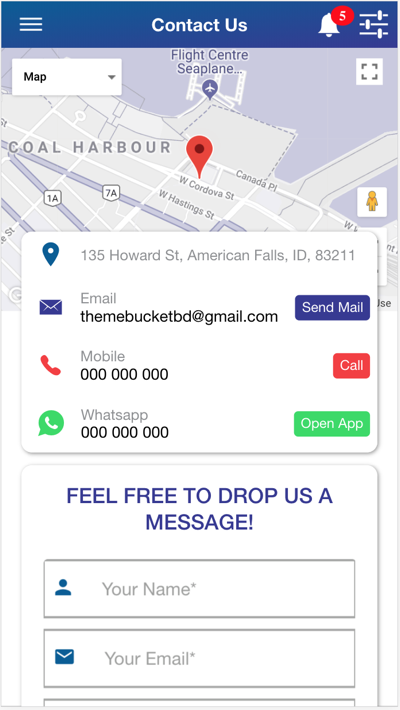The image is a screenshot from a contact us page on a mobile phone. It begins with a blue banner at the top bearing the text "Contact Us" in white. To the right of this text is a bell icon with a small red circle displaying the number 5, presumably indicating notifications.

Beneath the banner is an interactive map centered on a location indicated by a red marker labeled "Coal Harbor." The marker represents the business's physical location.

Superimposed over the bottom part of the map is the business address: 135 Howard Street, American Falls, Idaho, 83211. Directly below the address is the email contact, themebucketbd@gmail.com. The contact information also includes a mobile phone number and a WhatsApp number, both represented by strings of zeros, indicating placeholders.

Further down, in bold blue capital letters, is an invitation for the user: "FEEL FREE TO DROP US A MESSAGE." Below this invitation is a form with two rectangular fields; one labeled for the user’s name and the other for their email.

The overall layout clearly displays how users can contact the business, offering both visual and textual guidance for interaction.